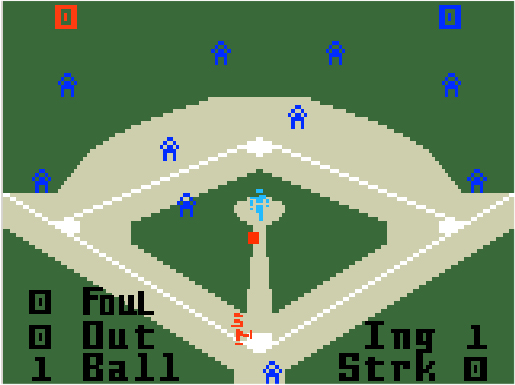This image is a screenshot of an extremely low-resolution, pixelated baseball video game from the late 1970s to early 1980s, likely from an Atari 2600 or Intellivision console. The game features a green baseball diamond with characters composed of simple, blocky pixels. The batter is represented by a red figure, and the opposing team, including the pitcher and fielders, is depicted in various shades of blue. In the top corners, the score is displayed as 0-0, with the red team on the left and the blue team on the right. Text overlays show the game status: zero fouls, zero outs, one ball, zero strikes, and it is the first inning. A small red square represents the baseball in play.